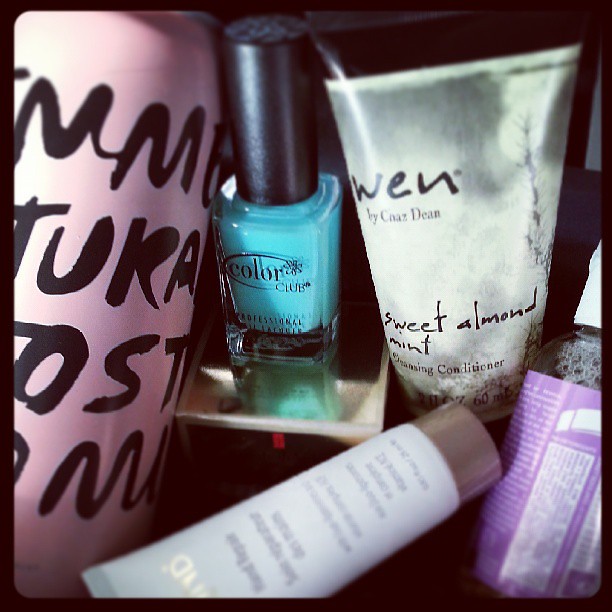This close-up image showcases an array of makeup products scattered on a dark, black or possibly gray marble surface. Prominently featured on the left is a pink tumbler-like container adorned with black, handwritten-style lettering, though the exact text is unclear. To its right, a small bottle of turquoise nail polish with a black cap is labeled "Color Club." Adjacent to the nail polish is a container of "WEN by Chaz Dean," labeled "Sweet Almond Mint Cleansing Conditioner." Further along, there's a white tube with a brown cap, likely a lotion, and beside it, a bottle featuring a purple and white label. The assortment of products and their varying shapes and colors create a visually intriguing composition.